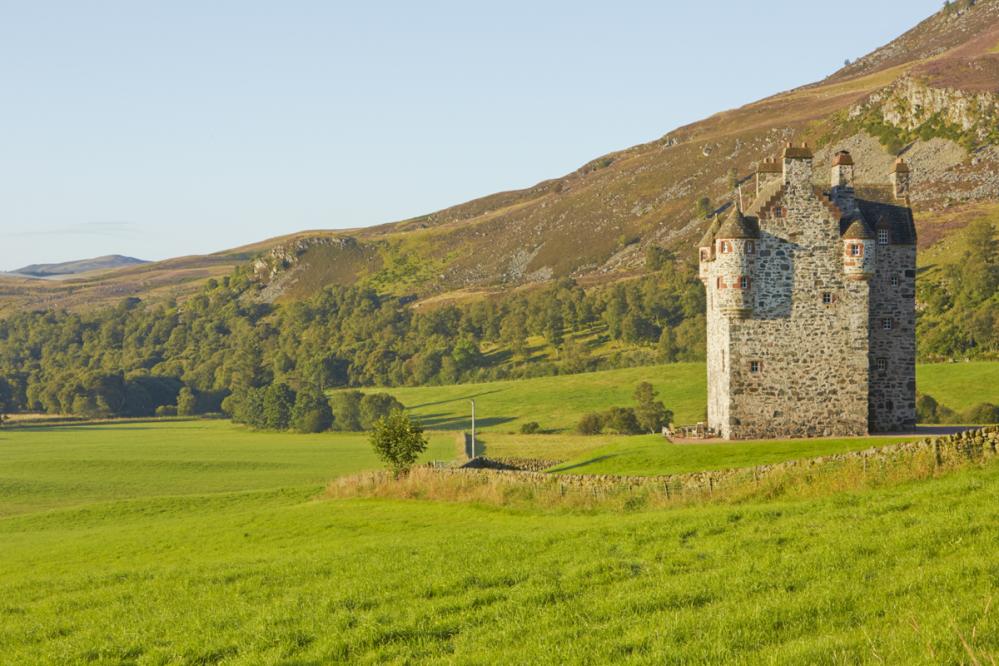The photograph captures a picturesque rural scene, featuring a modest yet striking standalone castle that resembles traditional Scottish and English manors. The castle, composed of grey and light brown stones, showcases classic architectural elements including turrets and tower-like structures at its hexagonal corners. It appears well-maintained, likely restored, and currently used as a residence. At least three stories tall, the narrow structure boasts several chimneys on its rooftop.

In the foreground, there's an inviting outdoor area with tables and chairs, suggesting a tranquil residential space. The castle is set amidst gently rolling hills covered in vibrant green grass, forming a lush meadow. The background reveals a dramatic landscape comprised of small mountains and a forested area, with a tree-lined slope that becomes steeper and rockier as it ascends to the top right. This steep hillside, devoid of vegetation, contrasts with the verdant surroundings.

The scene is bathed in sunlight under a clear blue sky, enhancing the vivid colors and serene beauty of the landscape. The absence of people in the photograph accentuates the peaceful, untouched nature of this charming rural setting.